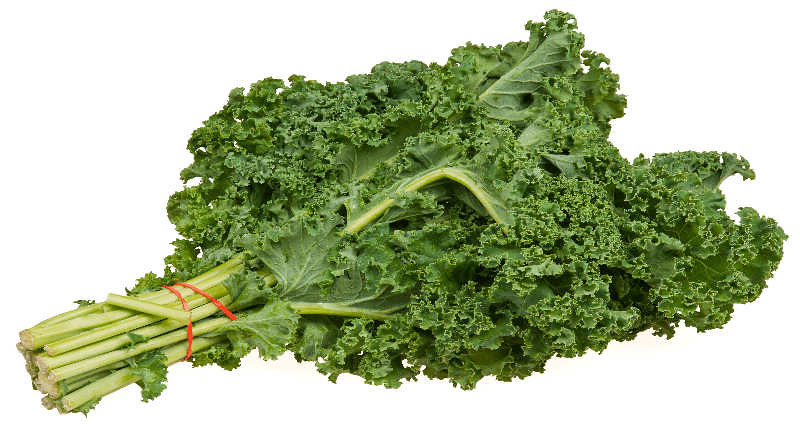This horizontal image features a fresh bundle of light green kale, tightly secured with a red rubber band wound around its cut stalks, which are about five inches long. The kale displays its trademark curly and fuzzy leaves, tapering to several points at the top. Notably, one of the long stems at the bottom is broken sideways but remains attached. The vibrant green leaves are prominent, some extending along the stalk with darker shades providing a contrast. The image is set against a plain white background, emphasizing the kale's fresh and crisp appearance, reminiscent of a grocery store purchase ready for salads.